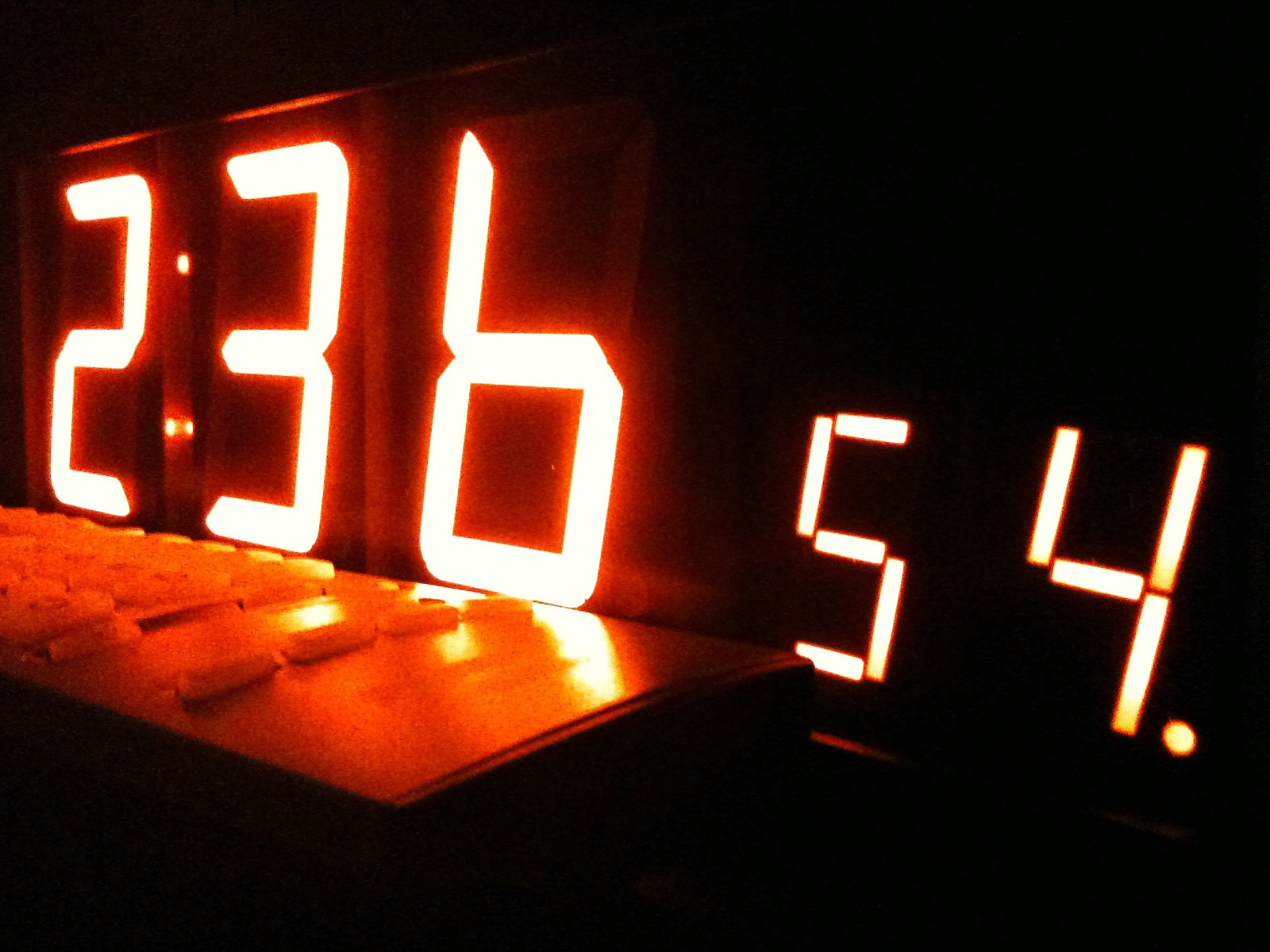The image depicts a digital clock display set against an entirely pitch-black background. The clock shows large, illuminated numbers "2:36" in the center, clearly indicating the time as 2:36. To the right of the time display, there are additional smaller numerals "54" followed by a dot, suggesting the seconds component, making the full time 2:36 and 54 seconds. In front of the clock display, there's an indistinct object which could be a keyboard or another item, resting on what appears to be a white table. The table has certain elements and buttons, though they are not distinctly visible due to the dark setting. The stark contrast between the bright clock digits and the pitch-black background draws the viewer's attention immediately to the time display, giving the image a dramatic, almost abstract quality.